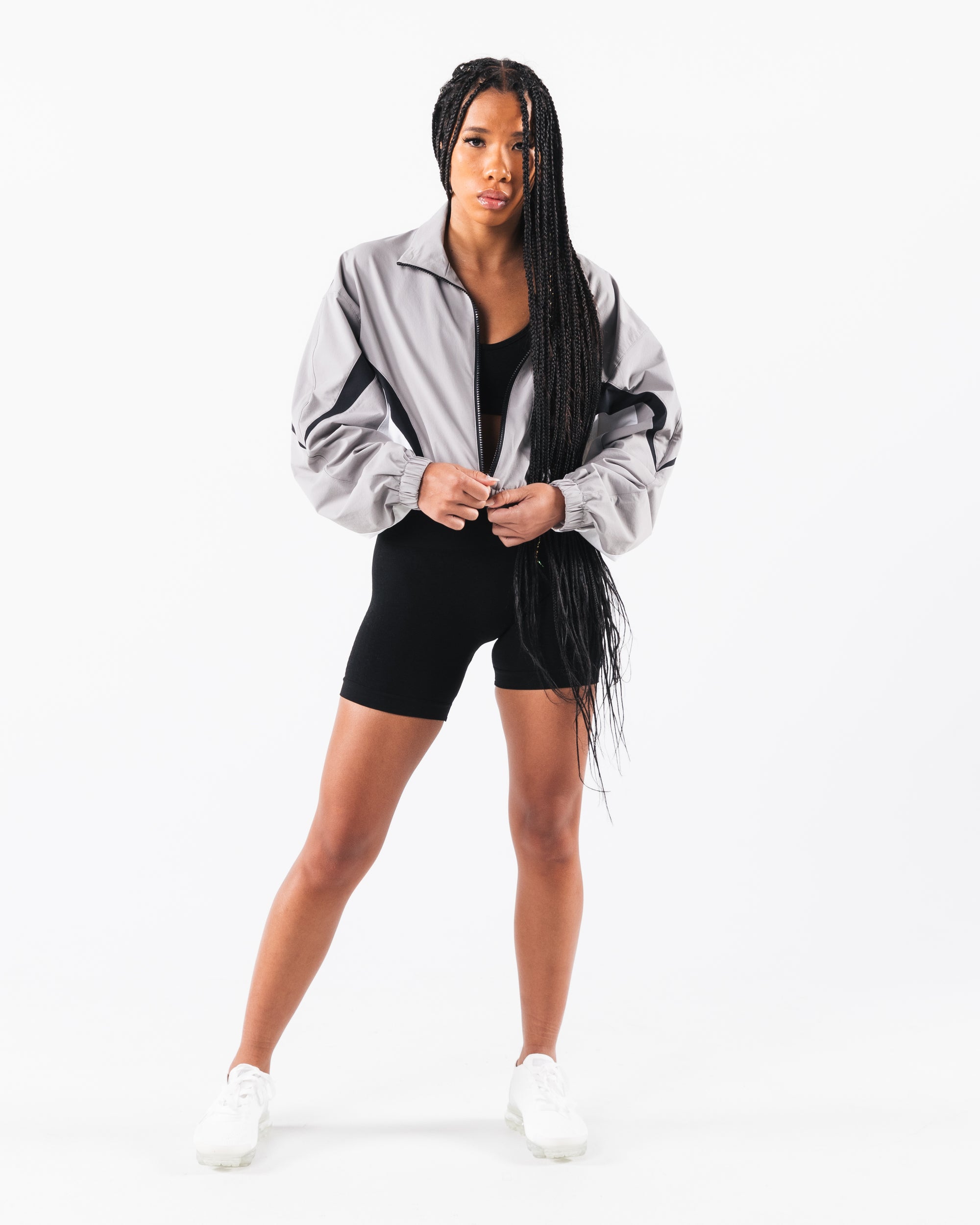The image features an African American woman who appears to be either a sports model or an athlete. She has very long hair, styled in numerous small braids that flow down past her waist, with some braids resting on her chest. She is dressed in a sporty ensemble consisting of black spandex pants and a white zippered sports jacket with black accents and a black zipper, which is unzipped down to her navel. Underneath the jacket, she wears a black sports bra. Her right leg is positioned slightly further apart than her left leg, and she is standing against a stark white background. The expression on her face is neutral or slightly sad, adding a sense of emotional depth to the scene.